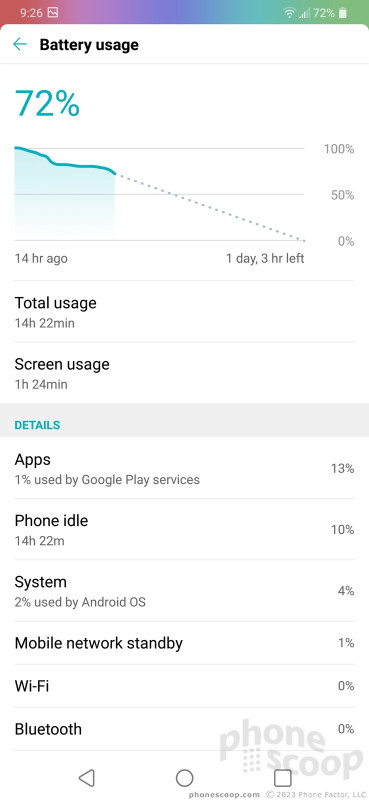**Image Caption:**

The image depicts a detailed breakdown of battery usage on a mobile device. At the top of the screen, there is a gradient bar indicating current battery levels, marked at 926 with a corresponding percentage of 72%. Below this, a graph visualizes the battery percentage over time, with markers at 100%, 50%, and 0%. The graph shows the battery level was nearly 100% 14 hours ago and has steadily declined since then, evidenced by a continuous downward slope and a diagonal dotted line.

A summary below the graph indicates that 1 day and 3 hours of battery life remain, with total usage recorded at 14 hours and 22 minutes. Screen time specifically accounts for 1 hour and 24 minutes of battery depletion. Further usage statistics reveal: 
- Google Play services consumed 13% of the battery,
- Phone idle time consumed 10%,
- The Android OS system consumed 2%,
- Mobile network standby used 4%,
- Wi-Fi and Bluetooth usage remain at 0%.

Additional design elements include a circle and a square icon, followed by the text "Phone Scoop." A backward triangle icon is also present. The primary text is black, while numerical and percentage values are highlighted in gray.